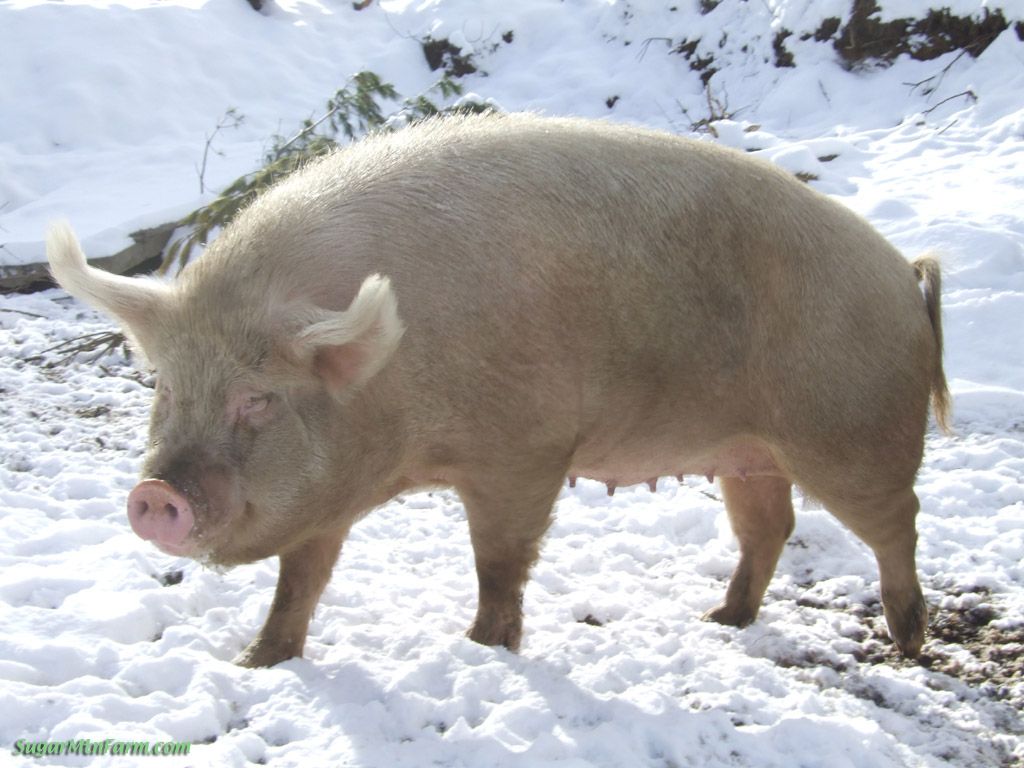A large tan pig with white-tipped ears and a pink snout stands in the center of a shallow, snowy field, taking up about two-thirds of the image. The snow is sparse enough to reveal patches of dirt and some vegetation poking through. In the background, there is a fallen tree or large bush covered in snow. The pig, which appears to be smiling slightly, looks toward the left of the frame. The image is stamped with a photobucket watermark, and there's a barely legible strip of text at the bottom due to its white transparency against the snowy backdrop. On the lower left, the website sugarloafarm.com is faintly visible.